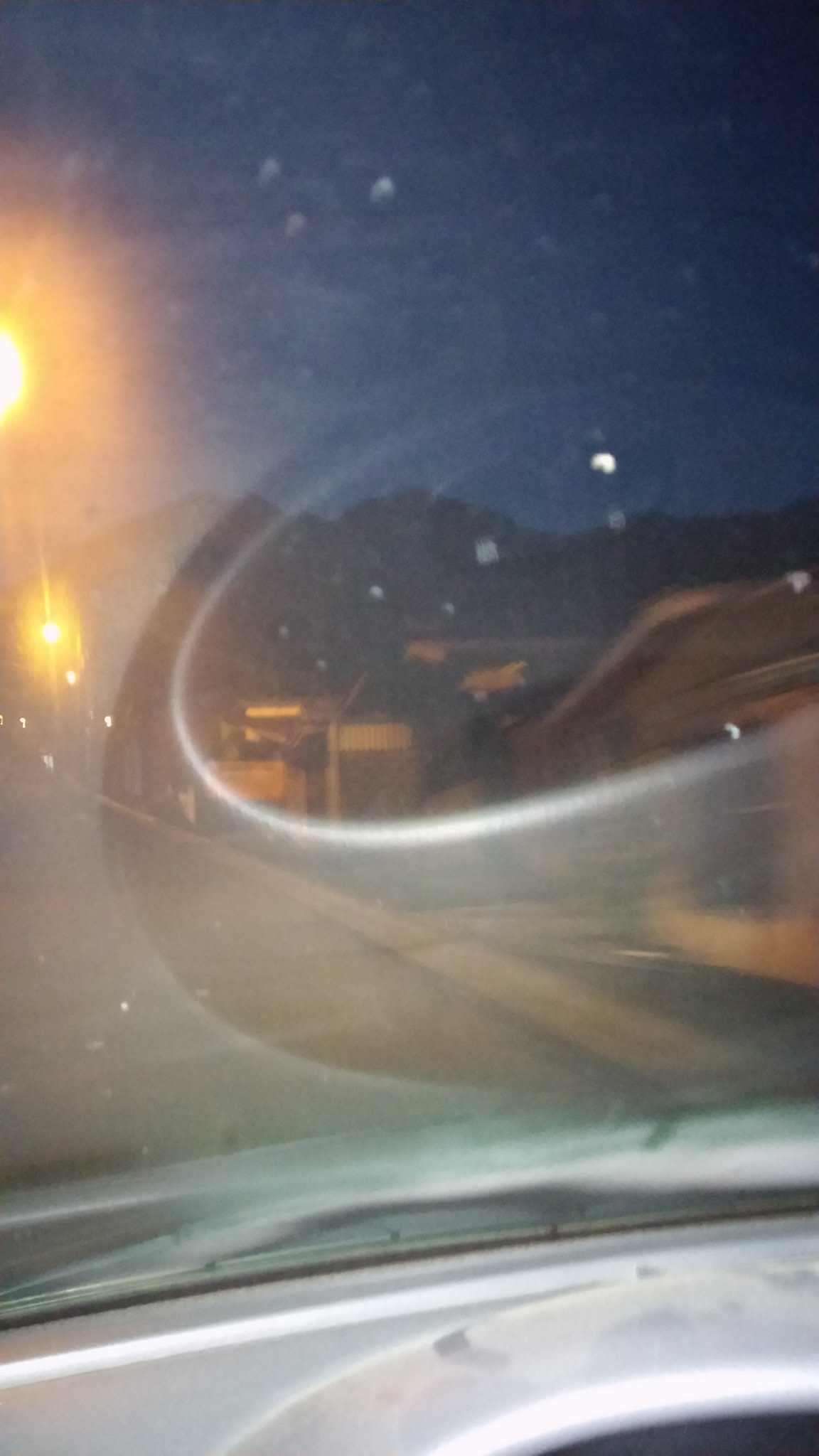This is an image taken from inside a moving vehicle, looking out through a windshield. It's dusk, transitioning into nighttime, casting a combination of dark blue and black hues across the sky. The lower part of the photo features part of the dashboard, adding a sense of depth and context. On the left side of the image, a couple of dispersed amber streetlights create a gentle glow, with one prominent streetlamp situated in the upper left corner. The right side of the image displays blurry silhouettes of houses and a possible sidewalk, indicative of motion blur from the moving car. In the distance, a shadowy mountain range looms against the faint evening light. Reflective patches on the windshield hint at interior elements of the car, contributing to the photograph's blurry and somewhat obscured view.